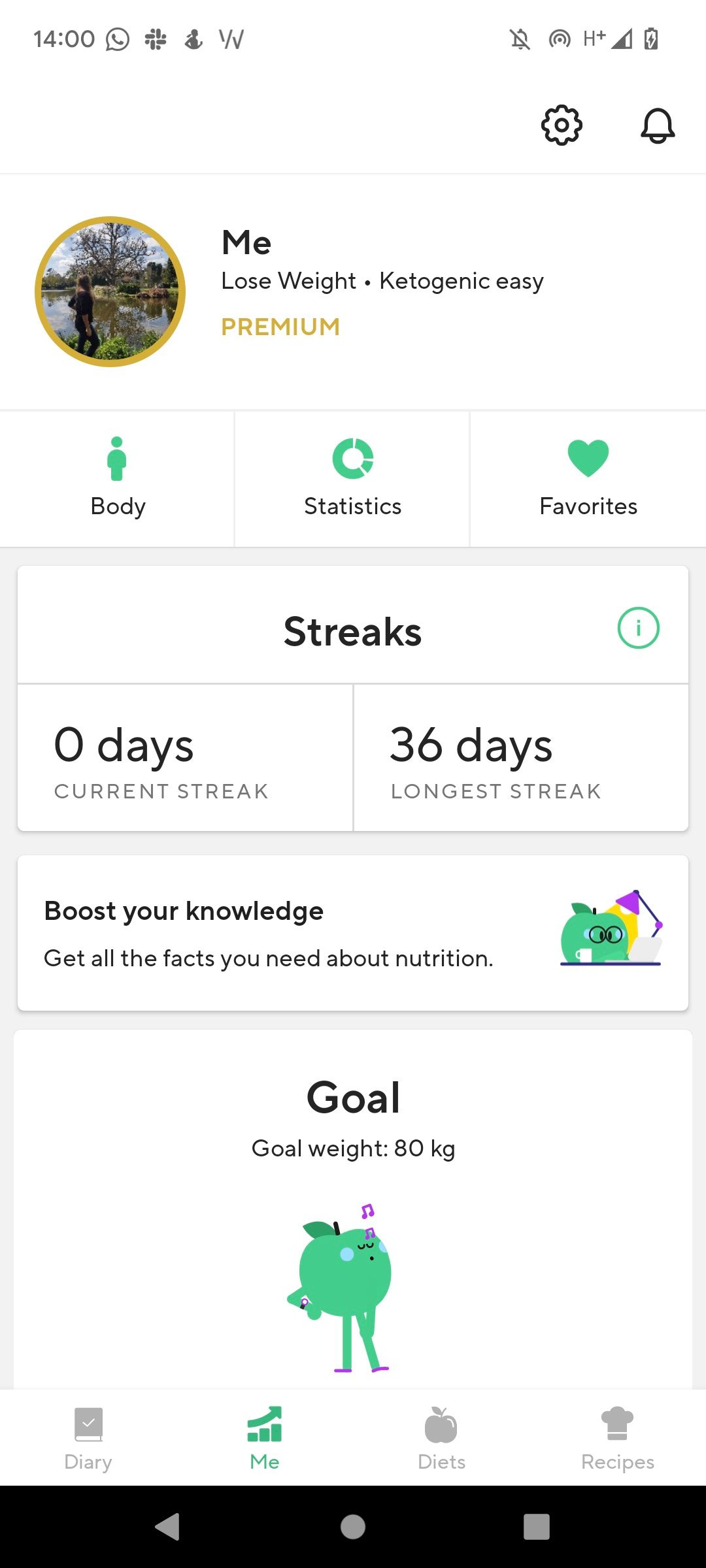This image displays a screenshot from a cell phone, with the time shown at 14:00 in the top left corner. Surrounding the time are some standard icons on both sides at the very top of the screen. Just below, on the top right side, there are a settings icon and a notification bell. 

Beneath these icons, there is a circular profile picture with a golden ring around it. The picture appears to depict someone standing on the edge of a pond with a tree in the background, and it is labeled "Me." Directly below the profile picture, there is text that reads "Lose Weight Ketogenic Easy." Further down, the word "Premium" is highlighted in gold.

Underneath this, a light gray horizontal line stretches from left to right, intersected by two vertical light gray lines. The vertical lines divide the space into three boxes. In the left box, the text "Body" is accompanied by a green silhouette of a person. The central box features the text "Statistics" next to an icon resembling a clock. Finally, the right box contains the text "Favorites" alongside a heart icon.